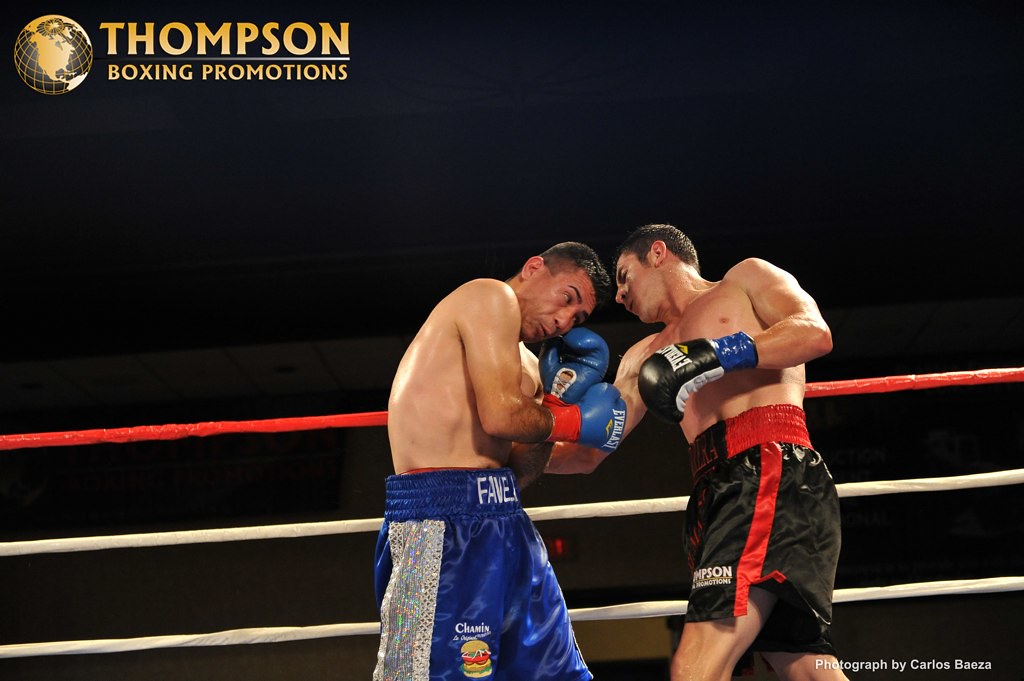The promotional image for Thompson Boxing Promotions captures an intense boxing match set against a stark black background. The top left corner features the company's name, "Thompson Boxing Promotions," in light gold lettering alongside a distinctive globe logo with grid lines but devoid of landmasses. The scene within the boxing ring is framed by red and white ropes, highlighting the action between two boxers from the knees up. 

On the left, a boxer clad in blue silk shorts, adorned with white letters spelling "Favel" on the waistband and a hamburger icon on the front, leans his head to the right. His attire includes gloves branded with either Everlast or Everblast. Opposite him, the boxer in black silk shorts with red stripes and matching black and white gloves seems to deliver a punch, his head tilting to the left. The image's primary colors—black, red, white, blue, and gold—are emphasized throughout the scene. 

In the bottom right corner, a watermark in white text credits the photograph to Carlos Baeza, adding another layer of professionalism to this gripping depiction of the sport.